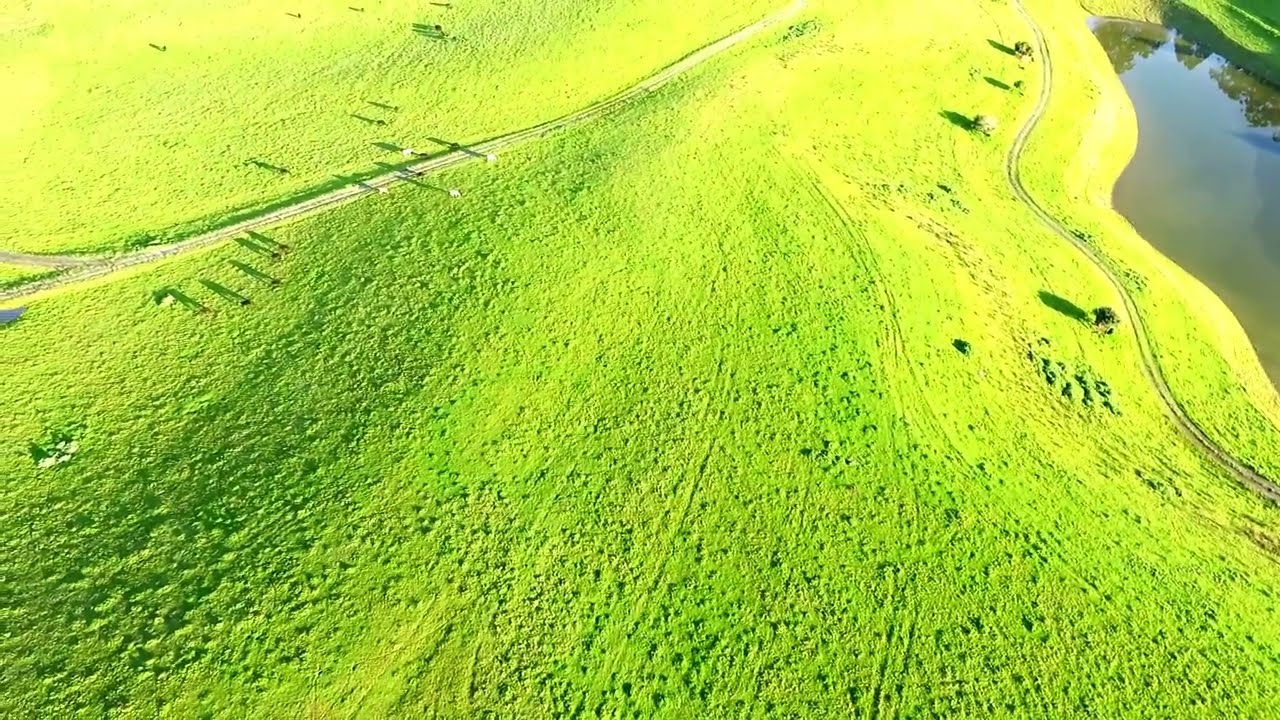This aerial photograph captures a vibrant, expansive countryside characterized by bright lime-green grassy fields with a yellowish tinge. The landscape includes a meandering white dirt and gravel road that winds through the fields, dividing into smaller one-lane paths at various points. The terrain gently slopes, forming a grassy hill, and the road appears to be tractor-made rather than for typical vehicular traffic. In the top left corner, a group of cattle—predominantly black and white, with a few brown—can be seen grazing. To the right of the image lies a small pond, possibly a rainwater reservoir, surrounded by a scattering of trees. The countryside is a picturesque, serene rural area, abundant with lush vegetation and pathways that bisect the verdant scene.